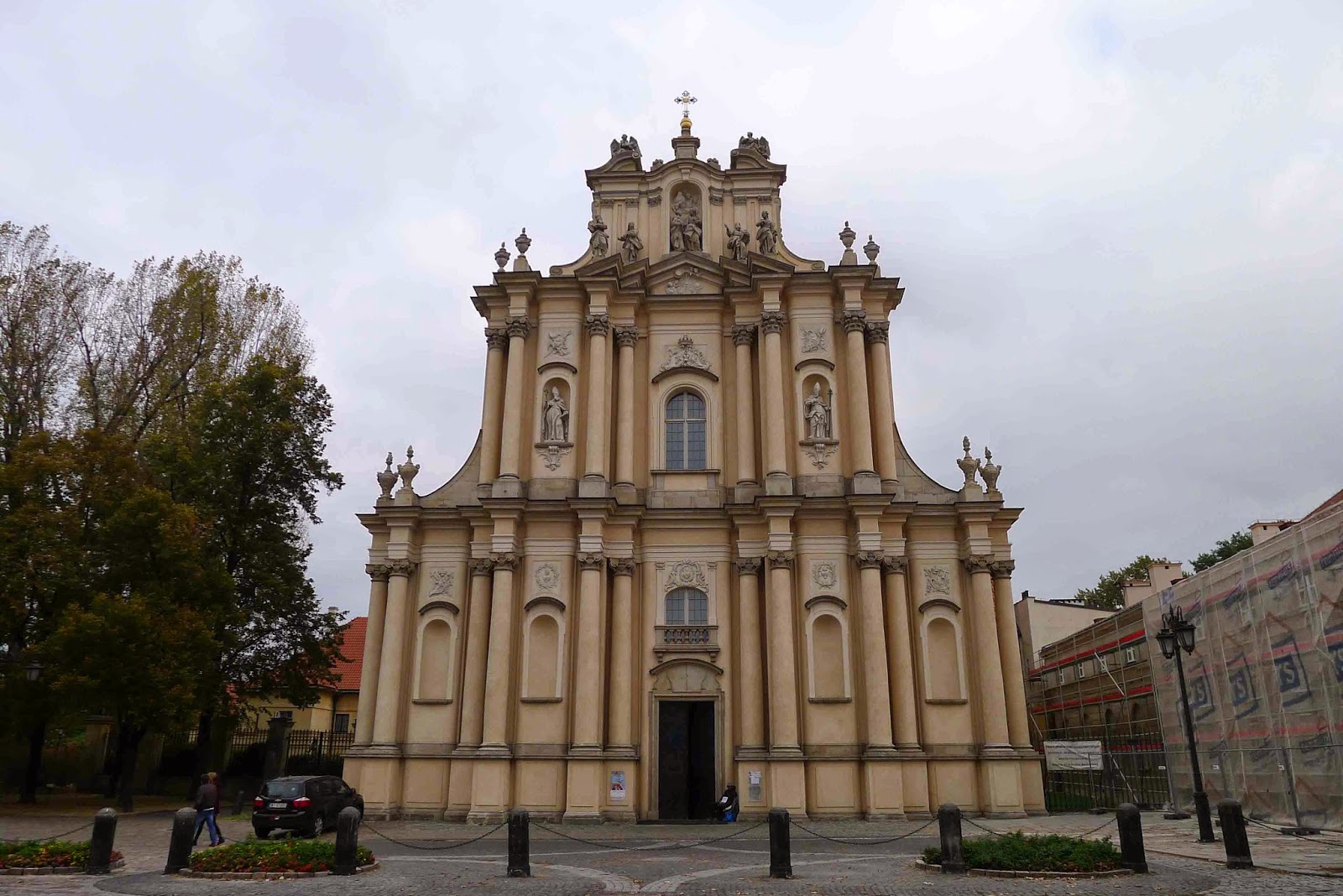The image is a horizontal, rectangular photograph showcasing a beautiful, traditional-style church made of pale, light brown concrete. The church, featuring an unusual architectural style suggesting it is located outside the United States, stands prominently in the center of the frame. It rises to three stories, crowned with a cross, and is adorned with statues of saints high up in the rafters. The church's facade boasts many columns and a grand, arched central front door, with multiple arched windows enhancing its old-world charm. 

The scene is set on a partly cloudy day, giving the photograph a somewhat dark tone, with the sky dominating the background. In front of the church, the pavement is sectioned off from traffic with pylons and chains. There is a small parking area in front, containing a car towards which a man is walking. Additional elements include a large tree on the left and several buildings on the right and behind the church, some of which are under construction. A red roof is also visible on the left side. Overall, the image captures the serene and historic ambiance of the church amid its urban surroundings.